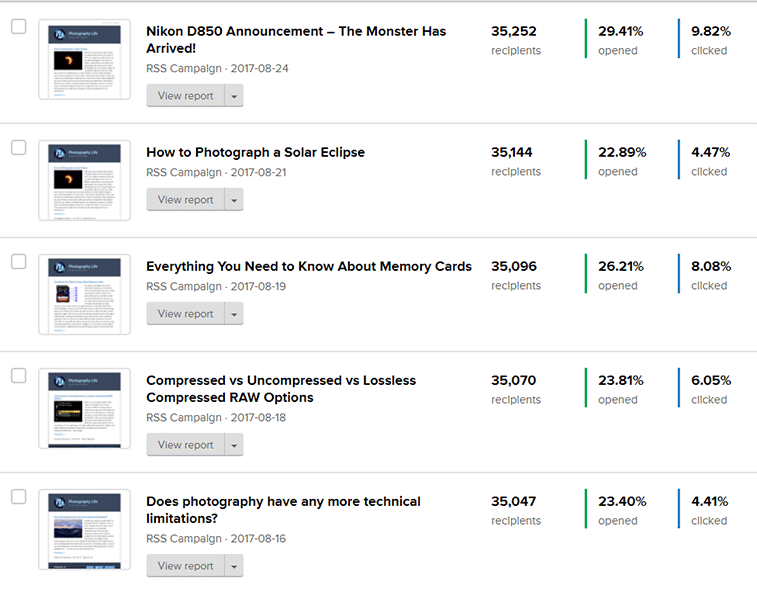The image depicts a series of editorial PDFs or newsletters, presumably for managing a subscription email list. These newsletters appear to be issued daily or every alternate day, with possible exceptions for weekends. The visual provides a snapshot of five distinct reports, with the latest one dated August 24, 2017. Each report has a unique title, including the most recent one, "Mekon D850 Announcement: The Monster Has Arrived." Detailed statistics accompany each report, showcasing metrics such as the number of recipients (35,252 for the latest), open rates (29.41% for the latest), and click-through rates (9.82% for the latest). The recipient count displays a slight daily growth, while the open rates remain consistently in the 20% range. Click-through rates fluctuate between 4% and 9%.